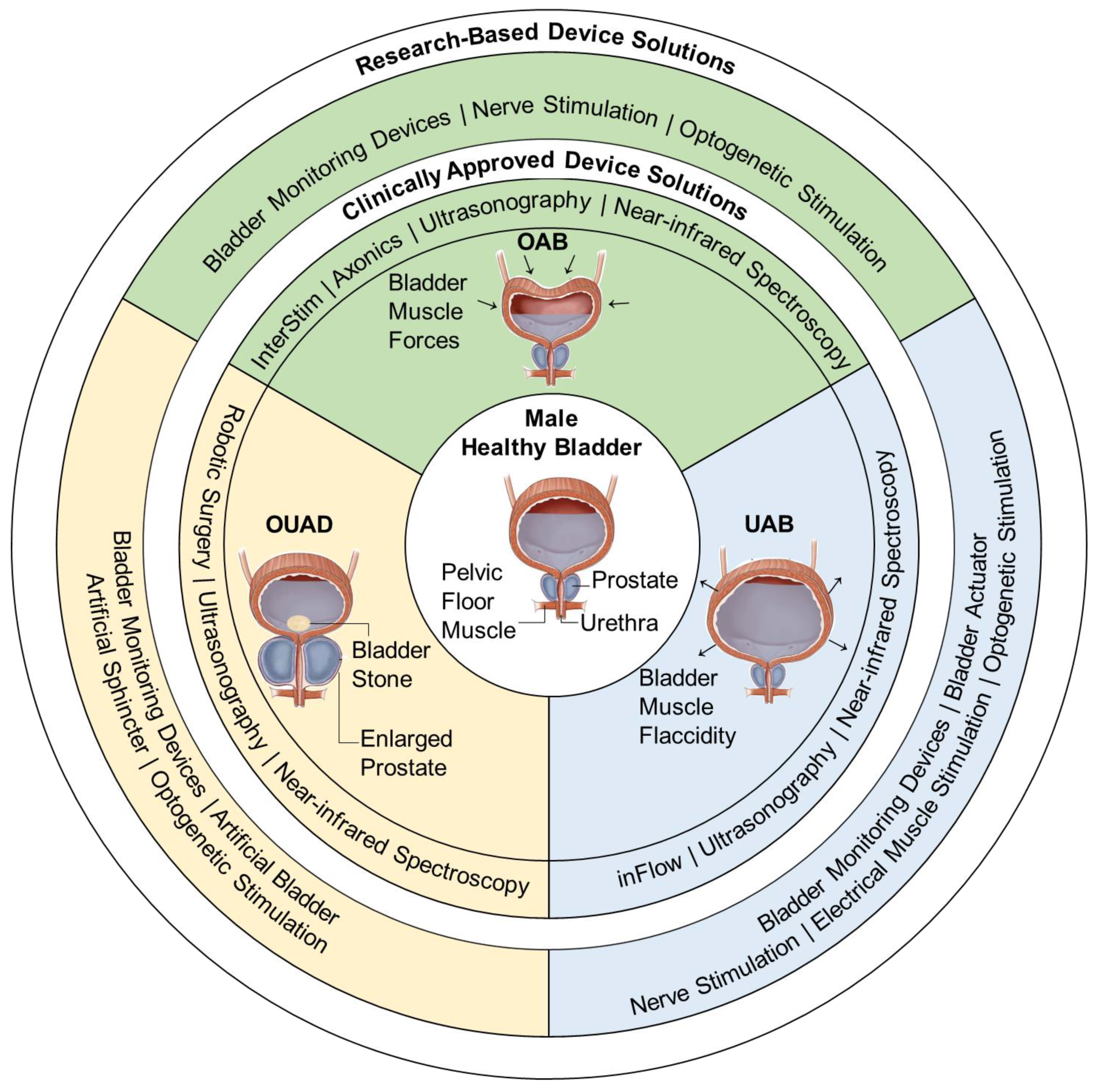This image is a detailed, circular medical diagram likely extracted from a medical text. It is divided into three equal segments, each representing different bladder conditions, all centered around a depiction of a healthy male bladder. The entire diagram is color-coded with black text and features a central white circle labeled "Male Healthy Bladder," depicting structures such as the pelvic floor muscles, prostate, and urethra.

The diagram's top third is highlighted in light green and labeled "OAB" (Overactive Bladder). This section discusses bladder monitoring devices, nerve stimulation, optogenetic stimulation, clinically approved device solutions, and lists items such as Innerstem, Axonics, ultrasonography, and near-infrared spectroscopy. It visually represents the bladder experiencing OAB.

Another segment is in light blue, labeled "UAB" (Underactive Bladder), and describes bladder muscle flaccidity. It also includes references to inflow, ultrasonography, near-infrared spectroscopy, bladder monitoring devices, bladder actuators, nerve stimulators, and electrical muscle stimulation, with a corresponding bladder image.

The third segment, in beige, is marked "QUAD" and focuses on bladder stones. It contains information about MICT (bladder emptying) and displays an image of the bladder with a stone. This segment also mentions the prostate's enlargement and various treatment methodologies such as robotic surgery, artificial bladder, and artificial sphincter.

Overall, this comprehensive diagram provides a visually rich and detailed overview of different bladder conditions alongside their respective monitoring and treatment devices.